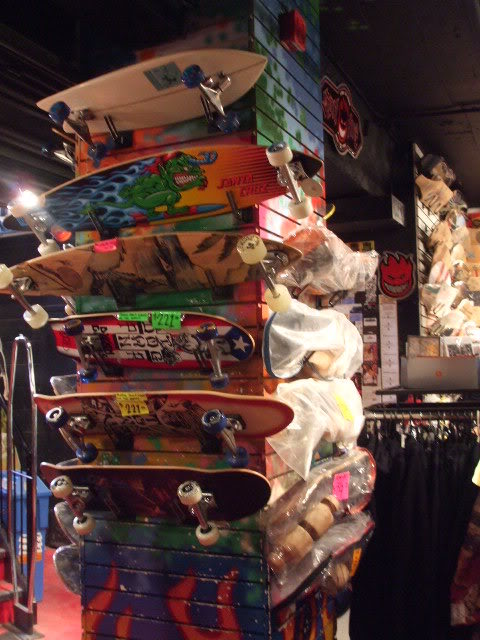The image captures the vibrant interior of a skate shop, featuring a tower-shaped wooden rack that ascends to the ceiling. This rack stands out with its eclectic paint job in colors like pink, blue, and green, adorned with flame designs and other whimsical details. The rack’s front is fitted with brackets holding six skateboards of varying sizes, each displaying unique and striking designs. One skateboard boasts an Evel Knievel-inspired pattern, while another features an orange backdrop with an indistinct green, possibly alien motif. A particularly notable board showcases the Puerto Rican flag and has a green price tag reading $221. The decks are adorned with colorful wheels in shades of black, blue, clear, and white.

The store’s backdrop reveals more about its layout; behind the skateboard rack, there are low clothing racks with black garments hanging on metal poles. The ceiling is painted black, with lights reflecting off the racks, adding to the shop’s edgy aesthetic. Additionally, a recognizable skateboard brand logo with a grinning, flame-haired face is visible, contributing to the store’s dynamic and visually engaging environment.